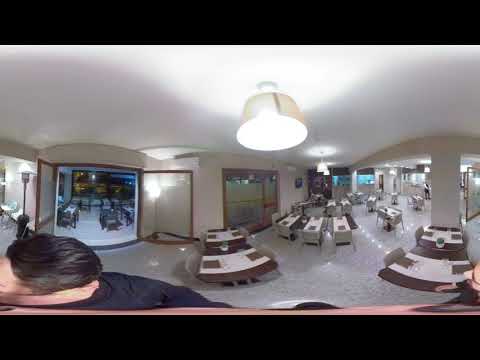The image depicts the interior of a bustling restaurant captured with a fisheye lens, providing a 360-degree view. Central to the image is a spacious dining area featuring approximately twenty brown wooden dining tables, each covered with pristine white tablecloths and set with two chairs. These tables are scattered rather than arranged in a strict pattern. The room is illuminated by a large, bright lamp hanging from the white ceiling, which complements the white walls and adds a sense of spaciousness.

On the left side of the image, there are double doors leading into another dining room with additional similarly-decorated tables. Next to these doors is a hallway. The floor features a white base with a textured black design, although the details are slightly obscured due to the blurriness of the photo. Along the right side, a kitchen area is visible through a doorway, discernible by a light blue light emanating from within.

Additionally, part of a man's head is visible at the bottom of the image; he is wearing a black shirt and has brown hair, presumably the photographer. The windows and other doors throughout the space have a wooden finish with glass panels, adding a touch of elegance to the overall design.